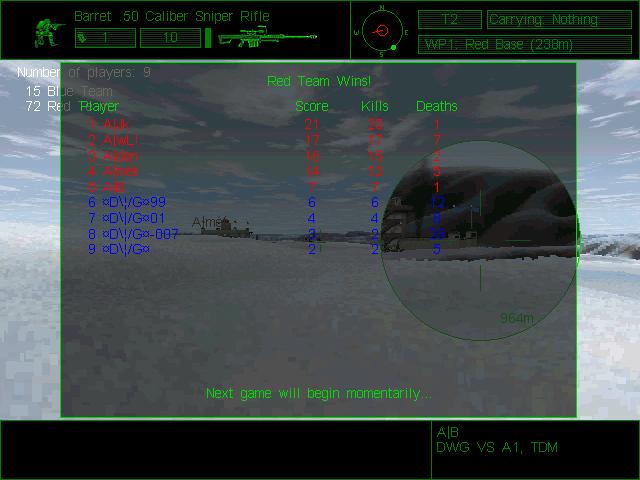The image depicts a victory screen from a video game, highlighting the conclusion of a team deathmatch between the Red Team and the Blue Team. Dominating the center of the screen is a bold green text declaring, "Red Team Wins." Below this, a notice states, "Next game will begin momentarily," indicating a brief intermission before the next match begins.

A detailed scoreboard is presented, divided into sections for the Red Team and the Blue Team, each listing nine players. The players' scores, kills, and deaths are displayed in respective team colors—red for the Red Team and blue for the Blue Team.

In the top right corner, a HUD element indicates the currently equipped weapon: a Barrett .50 caliber sniper rifle, with its ammunition count showing both the bullets in the gun and those held in reserve. Additional HUD information reveals that the player is positioned in the red base and facing west, as indicated by an on-screen compass.

At the bottom of the screen, text clarifies the game mode and teams involved with the inscription, "DWG vs A1 TDM," where TDM stands for Team Deathmatch.